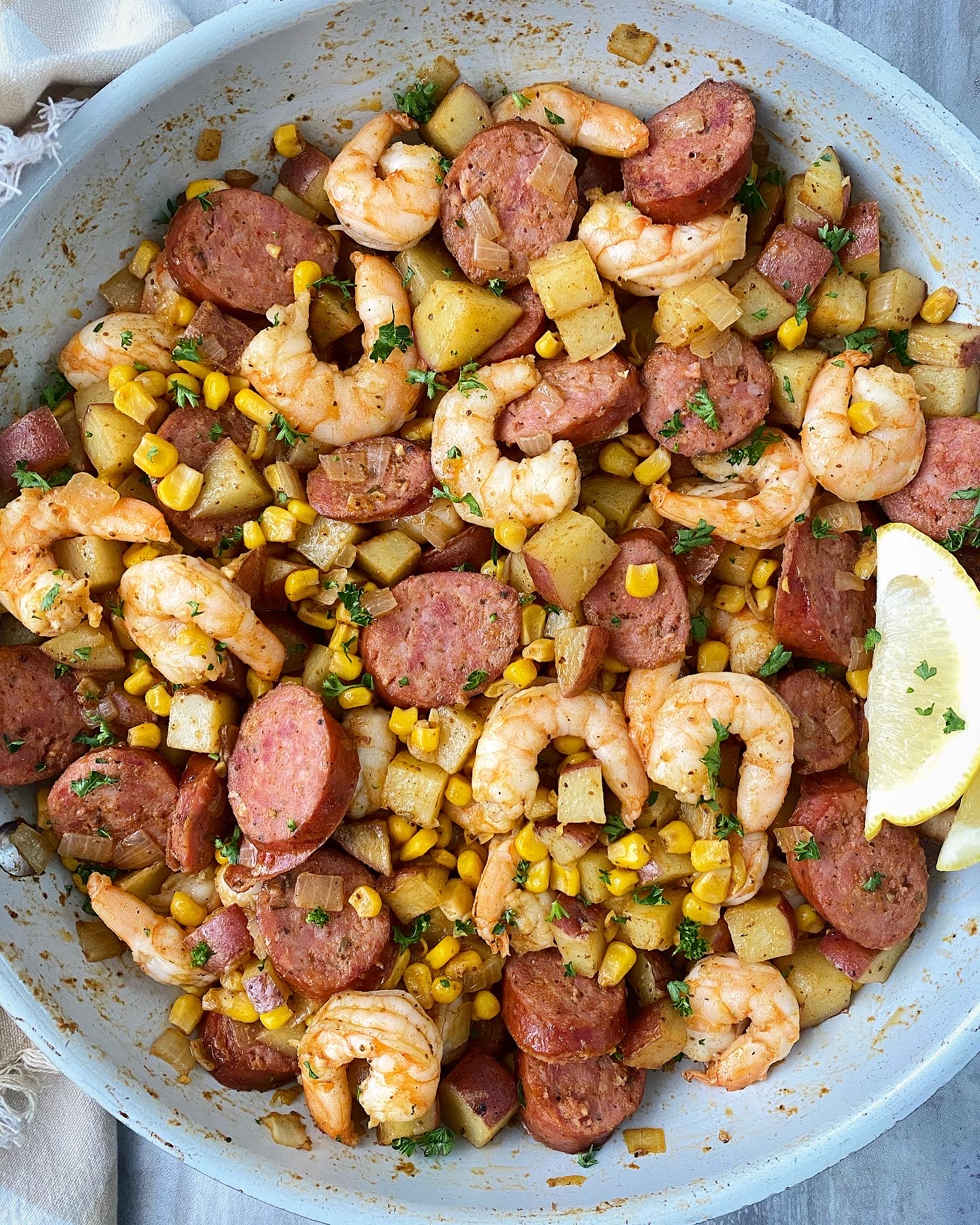The picture captures an overhead shot of a deliciously prepared dish presented in a large, light-colored bowl, possibly light blue or white enamel. The bowl, which appears to be plastic or enamel rather than glass, dominates the image, leaving only a small glimpse of the light blue wooden table it rests on, with some napkins nearby. The dish itself is a vibrant mix of ingredients: generous portions of sausage, shrimp, red potatoes cut into squares, small chunks of carrots and onion, and bits of corn. Everything is cohesively brought together with a sprinkle of fresh parsley or a similar herb, and the entire mixture is richly seasoned, possibly with a brownish-red sauce. In the center, there's a slice of lemon adding a fresh touch. The overall presentation is mouth-watering and looks like something straight out of a food blog, potentially as a header image for a recipe. The dish exudes a rustic, hearty appeal, reminiscent of a well-spiced Cajun hash.